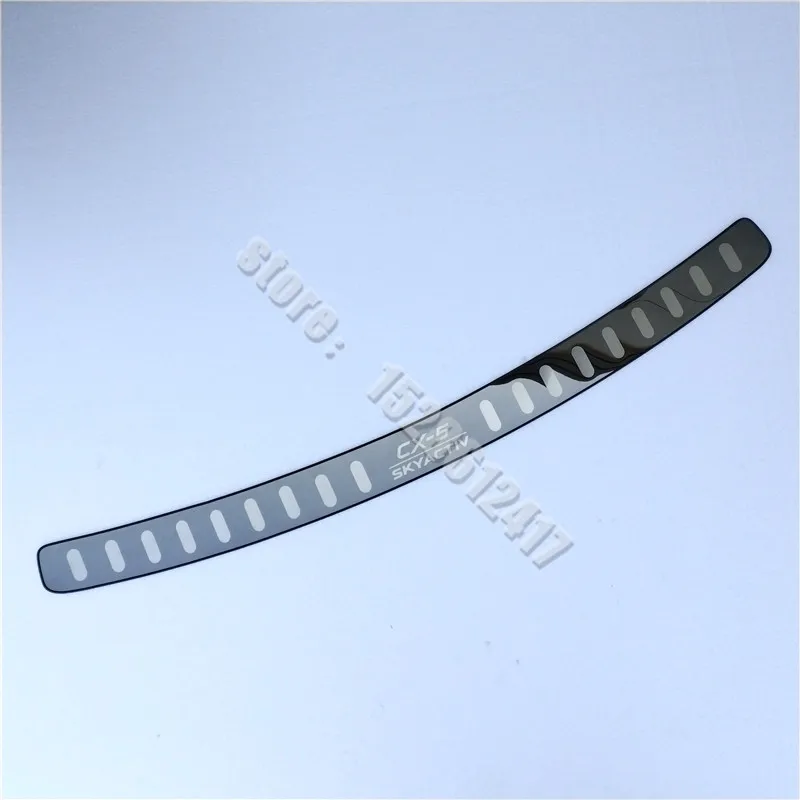This image features a distinctive black wristband set against a tranquil, light blue sky background. The wristband, which tilts slightly upward from the bottom left to the top right of the image, has a sleek, elongated rectangular shape with a darker black outline. Inside the wristband are several horizontal, pill-shaped cutouts that are lighter gray and slightly translucent. The center of the wristband prominently displays the letters "CX-5" underlined, with "SKYACTIV" written beneath in light blue capital letters. Overlaying the image is a diagonal watermark in white text that reads "store: 1528612417," starting from the top left corner and extending to the bottom right.